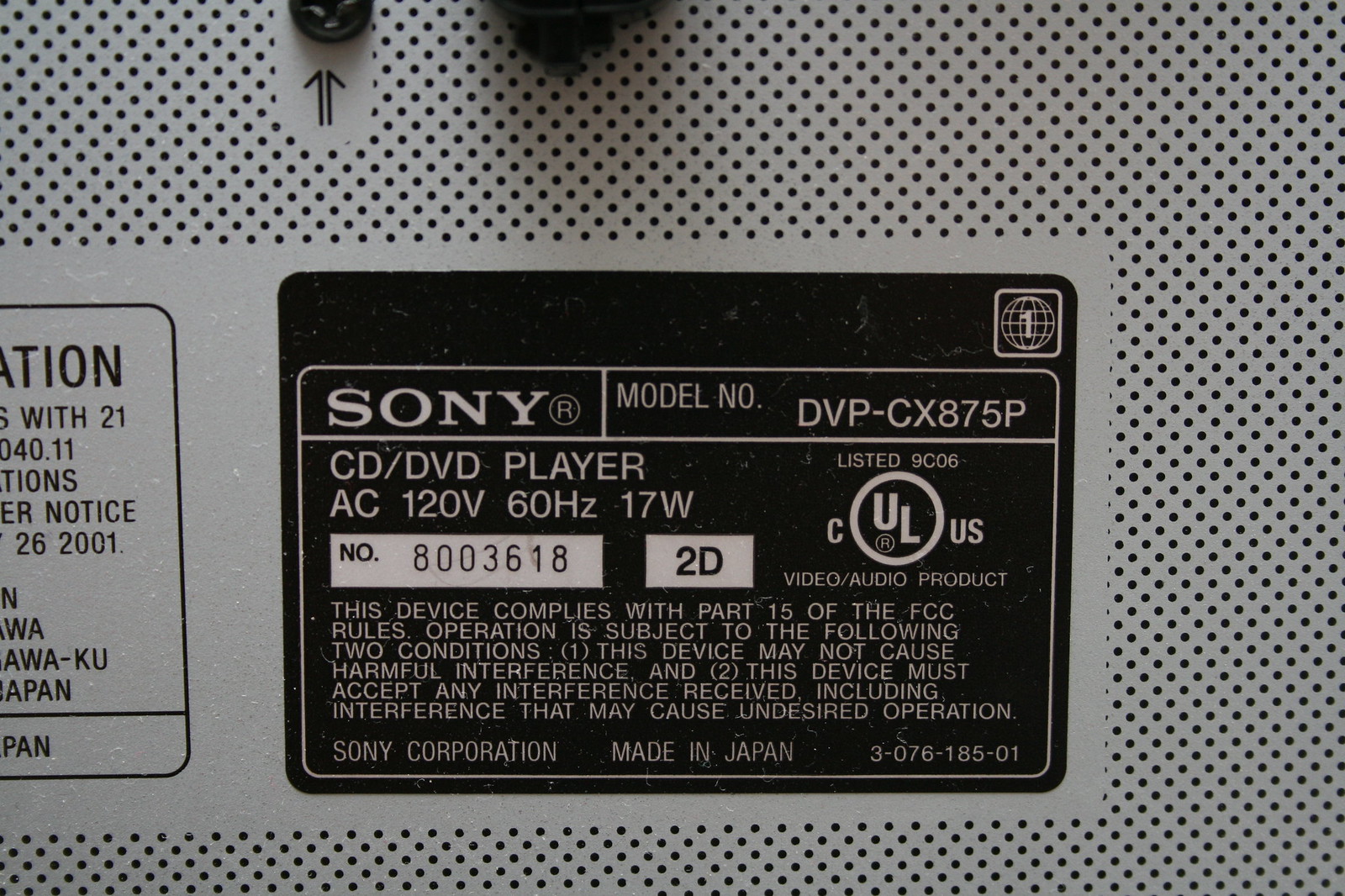This photograph captures the back panel of a Sony CD-DVD player, highlighting key information and its central label. The device, a model DVP-CX875P, features a vented, porous patterned metal surface, predominantly silver with black detailing. The central black badge prominently displays the white Sony logo on the top-left and the model number DVP-CX875P on the top-right, with the text "CD-DVD player, AC 120V, 60Hz, 17W" immediately below the Sony logo. There is also a white box labeled "No. 8003618" and "2D" on the black badge. Further details include the regulatory compliance statement: "This device complies with part 15 of the FCC rules. Operation is subject to the following two conditions: (1) this device may not cause harmful interference, and (2) this device must accept any interference received, including interference that may cause undesired operation." At the bottom of the badge, it states "Sony Corporation, made in Japan, 3-076-185-01." The overall image emphasizes the distinct contrast between the silver body and the black label, making the informative badge the focal point.